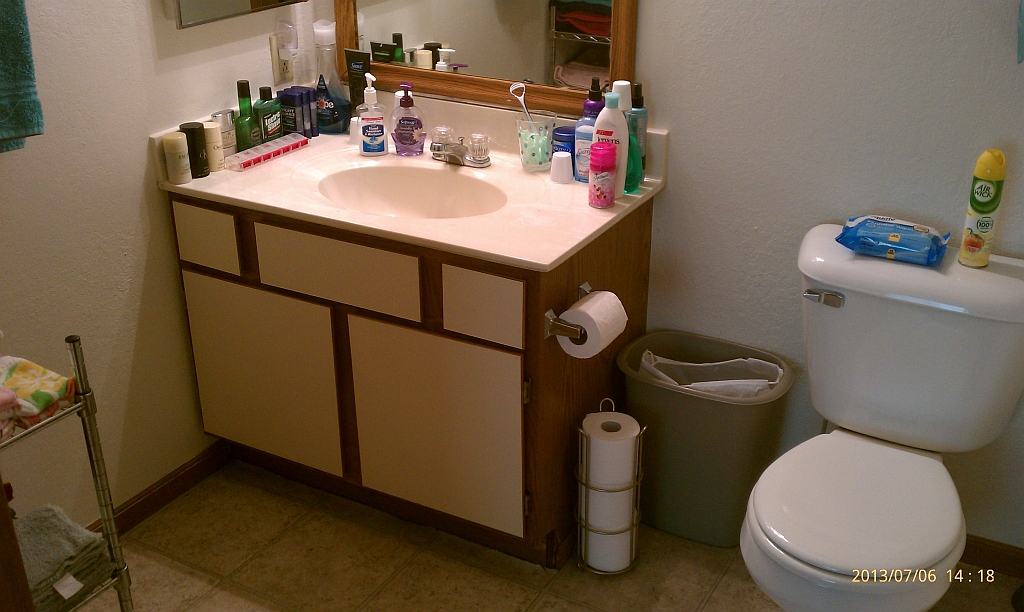A digital photograph captured in a bathroom showcases a pristine, white-tiled space on both the left and right sides. Dominating the right-hand side is a gleaming white toilet with the seat down. Perched on top of the toilet is a can of Airwick air freshener, distinguished by a yellow cap and a green design on a white base. The text "Airwick" in green is visible on the bottom right of the can. Notably, the toilet seat bears an inscription in yellow text that reads "2013/0706," followed by "1418" in white text.

The bathroom floor is composed of darker cream-colored tiles with matching grout. Positioned to the left of the toilet is a gray garbage can lined with a white bag. In front of the garbage can, some rolls of white toilet paper are stacked, revealing the off-brown cardboard insert of the topmost roll within a silver metal holder.

Adjacent to the toilet is a vanity unit with a wooden-colored base and white cabinet drawers. The lower section features two large drawers, while the upper section comprises three smaller drawers, with the central drawer being more rectangular. A toilet paper dispenser is affixed to the wall near the vanity, holding a roll of white toilet paper.

The vanity is topped with a white sink basin and a silver faucet positioned in the center, flanked by two clear handles. The countertop is cluttered with an array of bottles and products, predominantly white on the right side, with some green and blue items on the left. Above the sink, a mirror with a lighter brown frame hangs on the wall.

In the bottom left corner of the image, a silver metal shelf is visible, while in the upper left, a blue towel appears to be hanging, suggesting it is draped over an unseen holder or hook. This meticulously detailed depiction captures the essence of the bathroom's layout and contents.